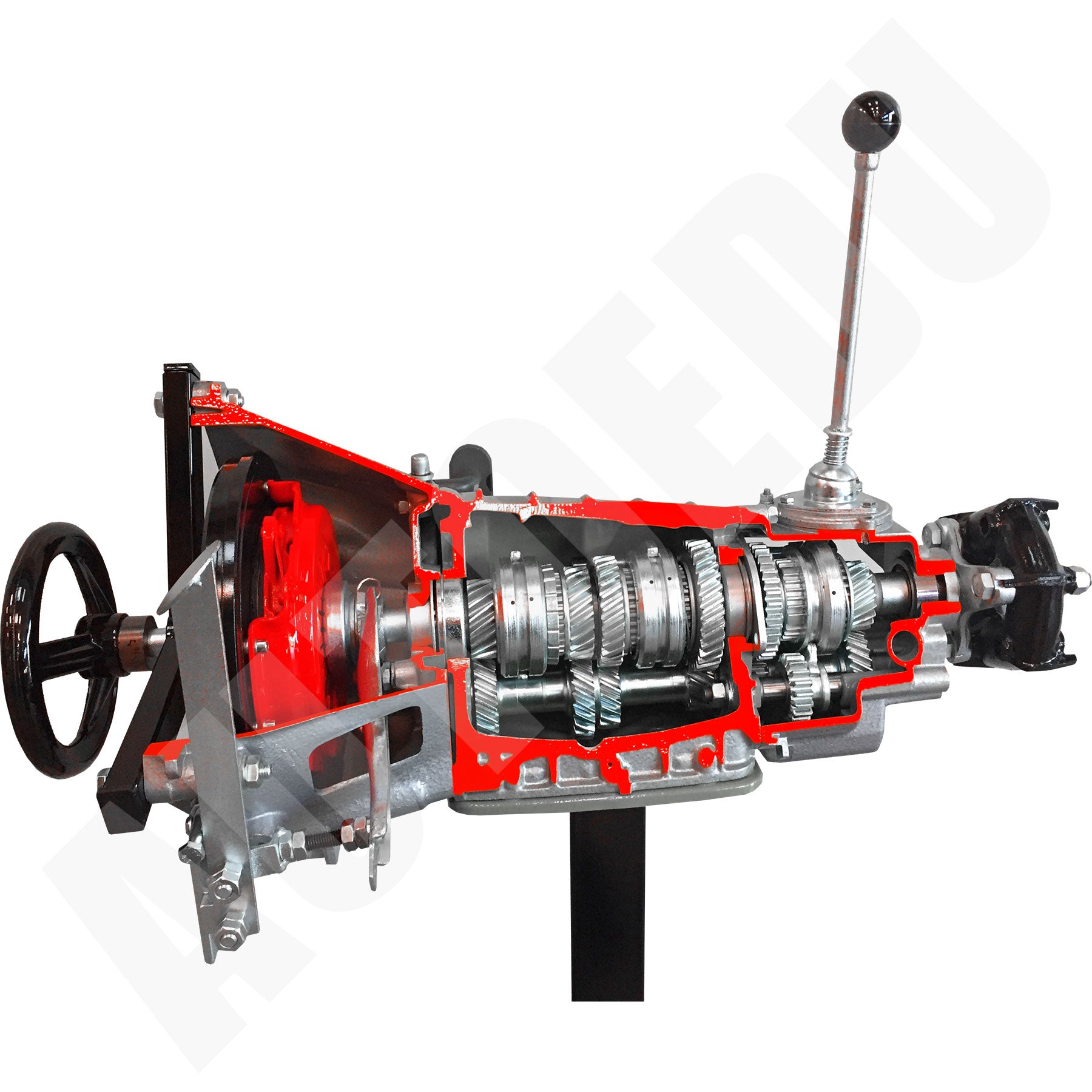The image depicts a detailed cutout view of intricate machinery, possibly a component of a larger system. On the left, there is a black turning valve connected to a piston mechanism, showing its function in controlling the machine. The unit exhibits a combination of silver, red, and black metallic parts, with the red framing highlighting certain sections. Throughout the device, various wheels, gears, and cogs with ridged edges are visible, becoming larger towards the center and smaller again to the right. At the top, a thin silver pole extends upwards, ending in a black spherical tip, resembling an antenna. Additionally, a black rectangular handle protrudes from the center downwards, and there are visible screws and bolts that suggest the machinery can be securely installed. A difficult-to-read watermark, likely representing the text "AUTOEDU," is present, indicating the image could be sourced from an educational textbook or diagram.